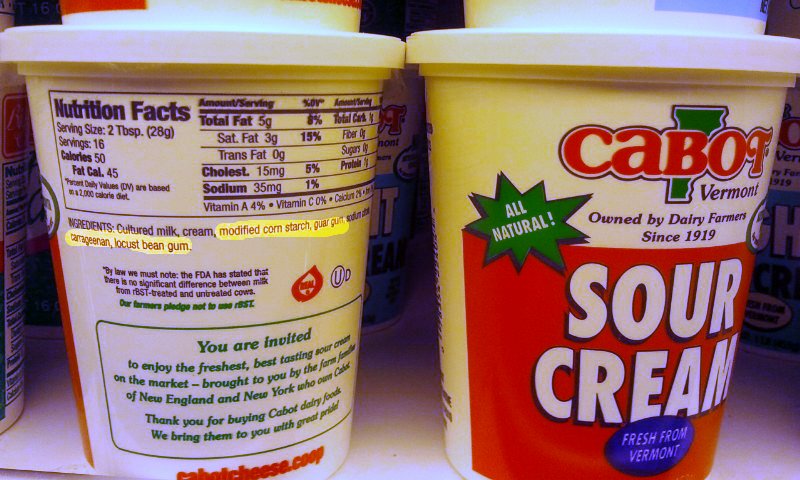This close-up photograph captures two containers of Kabat Vermont sour cream on a grocery store shelf. The containers are white and cylindrical with plastic lids. The left container is shown from the back, displaying the Nutrition Facts label, a list of ingredients, and a paragraph about the manufacturer, Kabat Dairy Foods. The text invites consumers to enjoy the freshest, best-tasting milk, and mentions that Kabat has been owned by dairy farmers since 1919. The right container, facing forward, features the brand's logo with the shape of Vermont outlined in green and bold red text that reads "Kabat." Below, in blue script, it says "Vermont." A red rectangle with white text declares "Sour Cream," while a blue oval states "Fresh from Vermont," and a green star highlights "All Natural". Additional containers of the same product can be seen in the background, reinforcing the setting as a grocery store aisle.